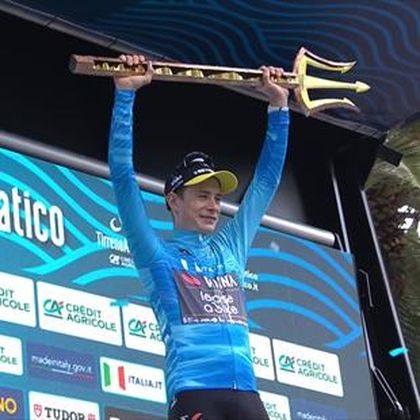In this detailed photograph, a very slender man is prominently standing center stage, holding a golden trident trophy aloft with outstretched arms. Clad in a form-fitting blue wetsuit-like outfit adorned with numerous sporting logos, indicative of sponsorships, he exudes athleticism and triumph. A baseball cap sits on his head, further accentuating his victorious stance. The backdrop features a board filled with an array of small, square logos from various companies, including Credit Agricole, suggesting a strong presence of advertising sponsors for the event. The setting appears to be an outdoor stage, likely under a structure with wavy lines on the ceiling colored in shades of dark and light blue, which adds a dynamic visual element to the scene. The colors throughout the image are vivid, with dominant hues including blue, yellow, gold, black, green, and red, providing a striking contrast to the man's figure and the celebratory atmosphere of the moment.